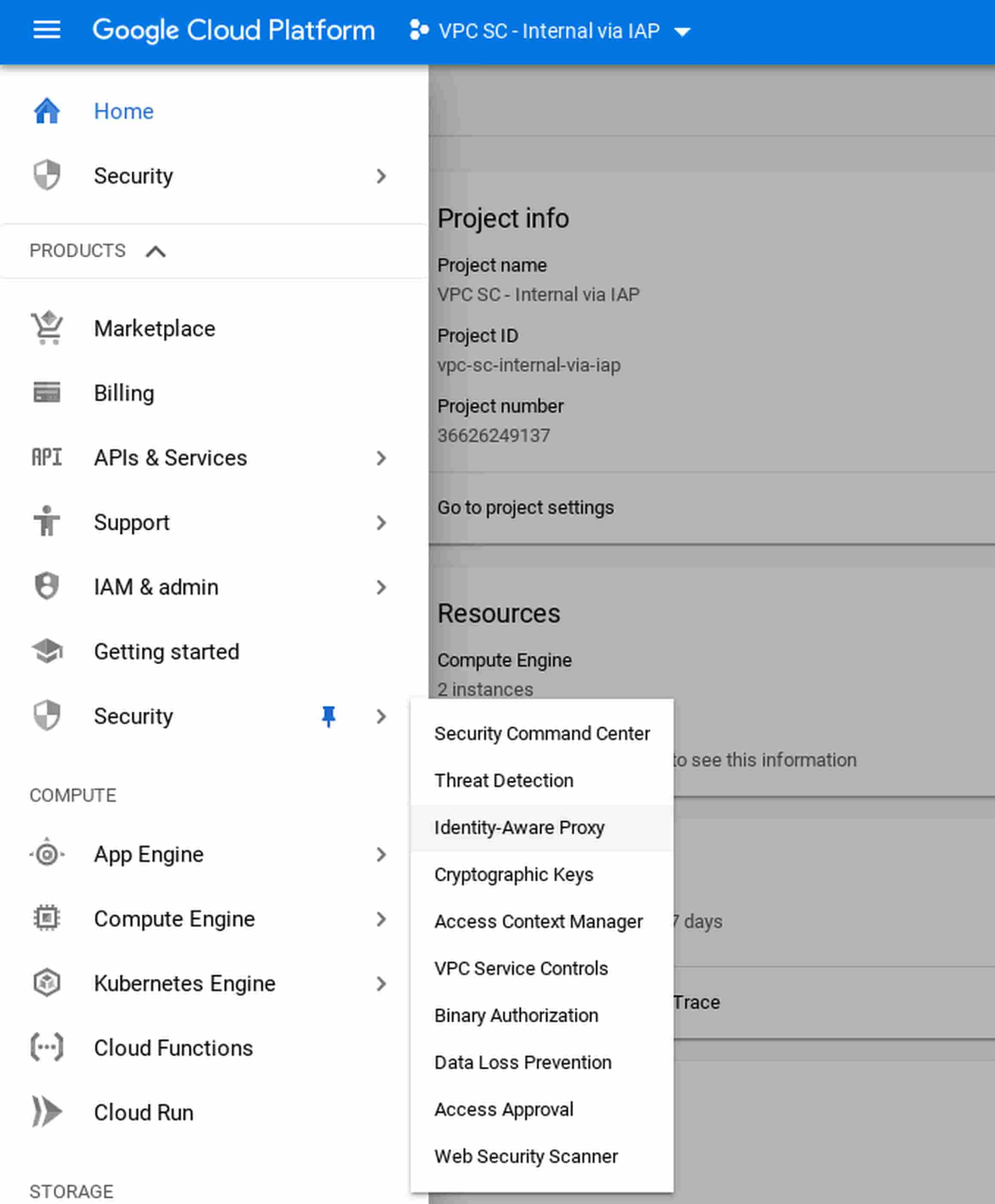The image features a dashboard interface of the Google Cloud Platform adorned with a blue banner at the top. On the left side of the banner, there are three horizontal white lines, next to which is the text "Google Cloud Platform" in white. Directly below this banner, there is a clickable drop-down menu labeled "VPCSC, internal via IAP."

The left side of the interface showcases a white-bordered sidebar menu that lists various navigational options: Home, Security, Products, Marketplace, Billing, APIs and Services, Support, IAM, Admin, Getting Started, Security, App Engine, Compute Engine, Kubernetes Engine, Cloud Function, Cloud Run, and Storage. Within this sidebar, the "Security" tab is expanded, revealing sub-options such as Security Command Center, Threat Detection, Identity-Aware Proxy, Cryptographic Keys, Access Context Manager, VPC Service Controls, Binary Authorization, Data Loss Prevention, Access Approval, and Web Security Scanner.

On the right side of the image, set against a gray background, there is a section titled "Project Info." This section details the project name "VPCSC, internal via IAP," project ID "VPC-SC-internal-via-IAP," and project number "36626249137." Additionally, there is a link that says "Go to project settings."